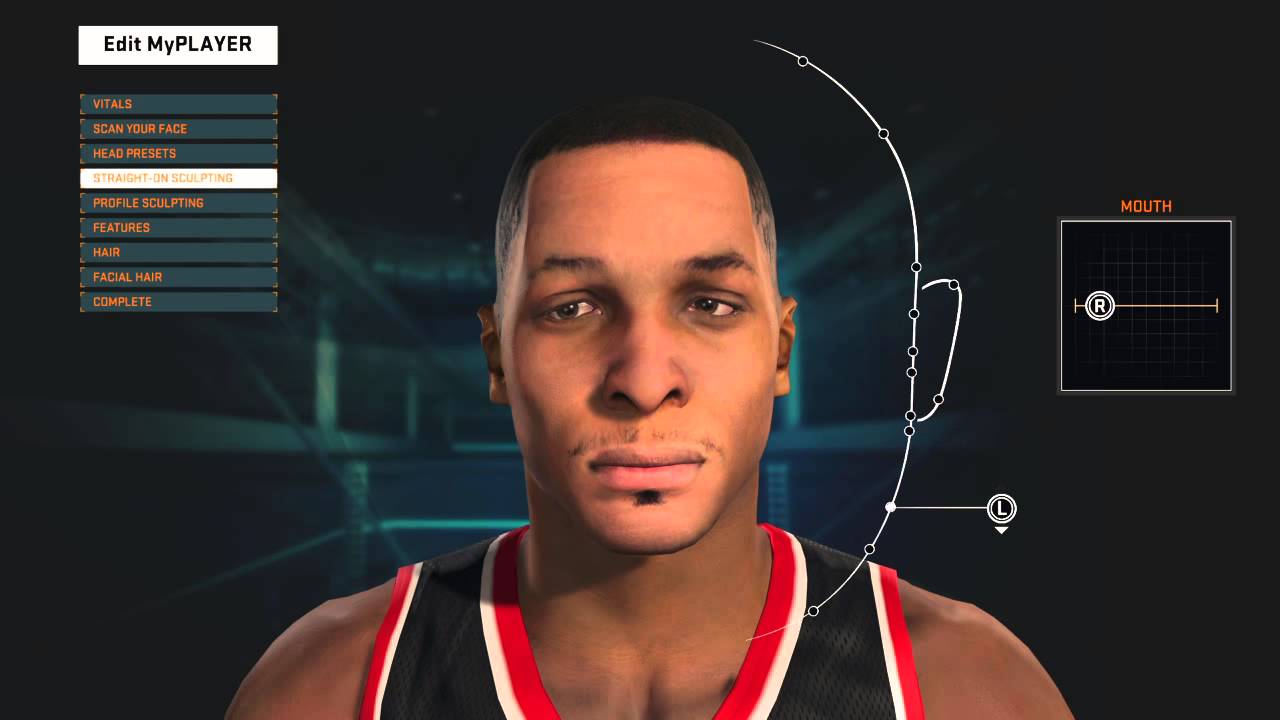The screenshot features a predominantly black background with a white box labeled "Edit My Player" in the upper right corner. Directly beneath this box is a vertical menu with various selection bars that read: "Vitals," "Scan Your Face," "Head Presets," "Straight-On Sculpting" (highlighted), "Profile Sculpting," "Features," "Hair," "Facial Hair," and "Complete."

At the center of the screen is an AI-generated illustration of an athlete, likely a basketball player. The figure has dark skin and is dressed in a dark navy blue tank top with a red and white striped border. The athlete's eyes are directed forward, and the mouth is closed, conveying a neutral expression. 

On the left side of the screen, there is an outline of a side profile of a face, an additional interface element to guide the sculpting options. Below this outline is a box labeled "Mouth," indicating this section is currently being edited. The screenshot appears to show an intricate interface used for customizing the physical characteristics of a virtual player.